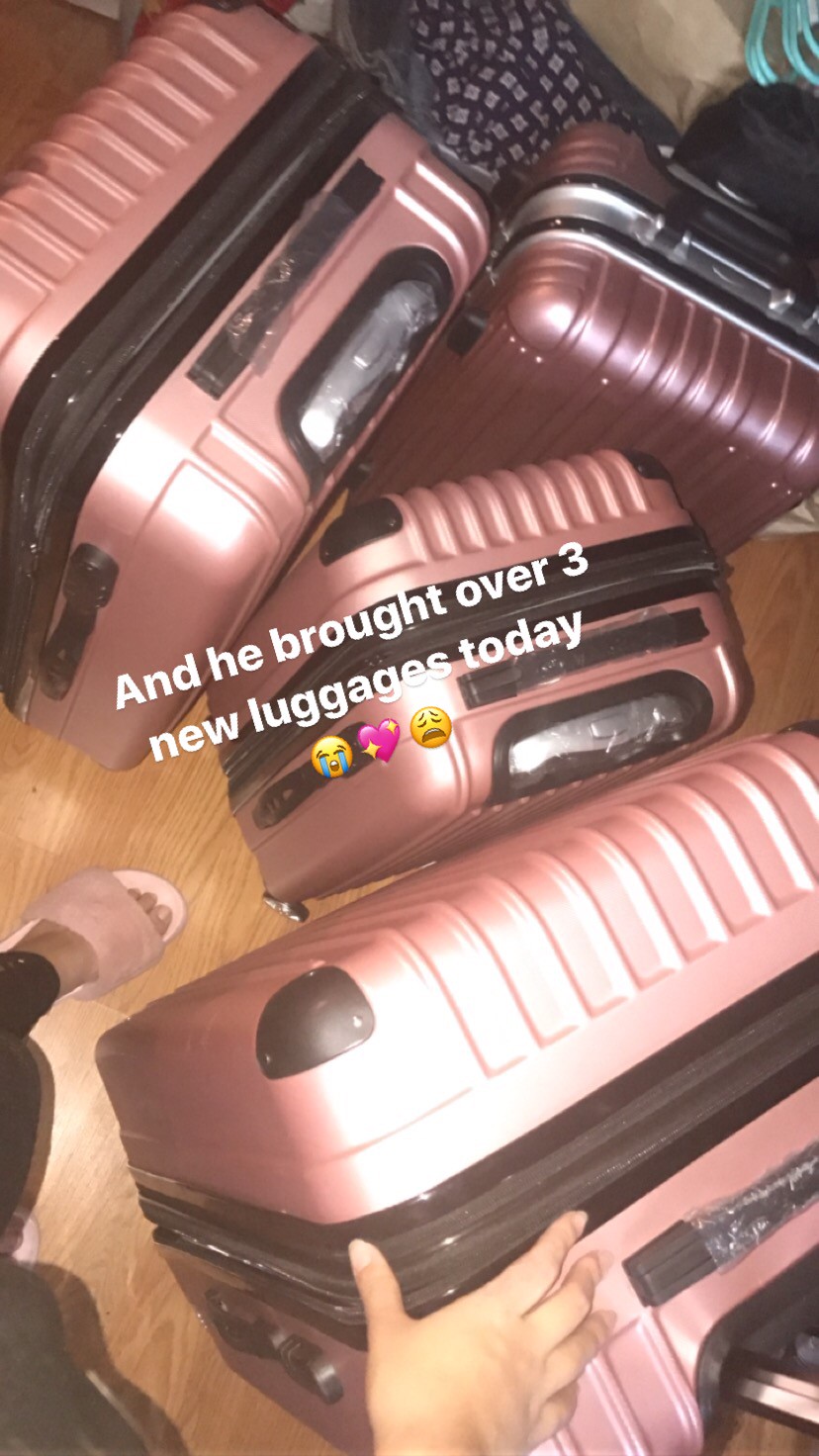In this image, we have a top-down view of four pink rollaway suitcases scattered across a light-colored wooden floor. The suitcases are of a regular pink shade, featuring black trim around the zippers and handle casings. The handles themselves are silver. The text "Andy bought over three new luggages today" is overlaid in the center of the image, accompanied by three emojis: a crying face, a heart, and an exhausted face.

A woman's hand, possibly her right hand, rests on one of the suitcases in the bottom right corner. She is wearing black leggings and pink slippers. Visible in the bottom part of the image is her left foot. Additionally, there is a noticeable blue fabric with white designs in the top part of the image, as well as a cyan-colored rope or hangers in the top right corner. The suitcases are positioned in a jumbled, scattered manner, enhancing the casual, slightly chaotic feel of the scene.